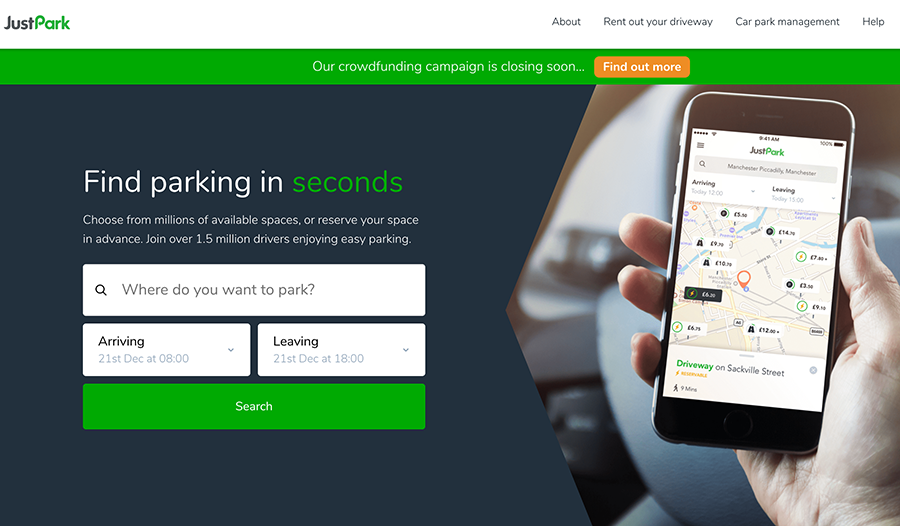The screenshot showcases the Just Park website, organized into three main sections. 

At the top, there is a navigation bar with a white background featuring the website name, "Just Park", and options to the right: "About," "Rent Out Your Driveway," "Car Park Management," and "Help."

Below this, a single-line high bar with a green background highlights an important announcement: "Our crowdfunding campaign is closing down soon," accompanied by a call-to-action button labeled "Find out more."

The main area of the screen, occupying the majority of the display, has a gray background and is dominated by an image of a person holding a smartphone displaying a map, which signifies the Just Park application in use. The left half of this section features the prominent title, "Find Parking in Seconds," and a subtitle promoting the service: "Choose from millions of available spaces or reserve your space in advance. Join over 1.5 million drivers enjoying easy parking."

At the bottom of this section, there is a search interface where users can input their desired parking location. Below the search box are two drop-down menus labeled "Arriving" and "Leaving" for specifying times. Finally, a green background button labeled "Search" is available for users to execute their search query after entering the required information.